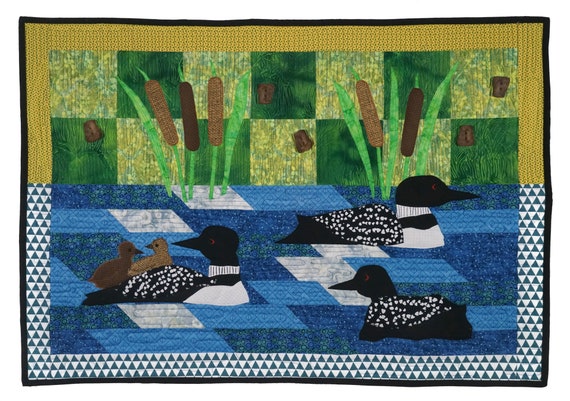This is a detailed and intricate handmade quilt, bordered in black, and divided into two distinct sections. The upper half is framed with a yellow stitched border and features a cross-section pattern of light green and dark green squares, emulating a ground-like area. Grass-like water reeds with cattails are intricately stitched, extending into this section, adding texture and depth. The lower half is bordered by a geometric pattern of alternating small blue and white triangles, resembling water. Within this blue quilted area, there are dark blue, light blue, and white splotches, creating a sense of movement and fluidity. Swimming in this water representation are three finely detailed black and white ducks with red eyes and pointed beaks. The duck on the far left carries two brown chicks on its back, looking in opposite directions. Two ducks are facing left while the third is facing right, adding a dynamic interaction within the scene.